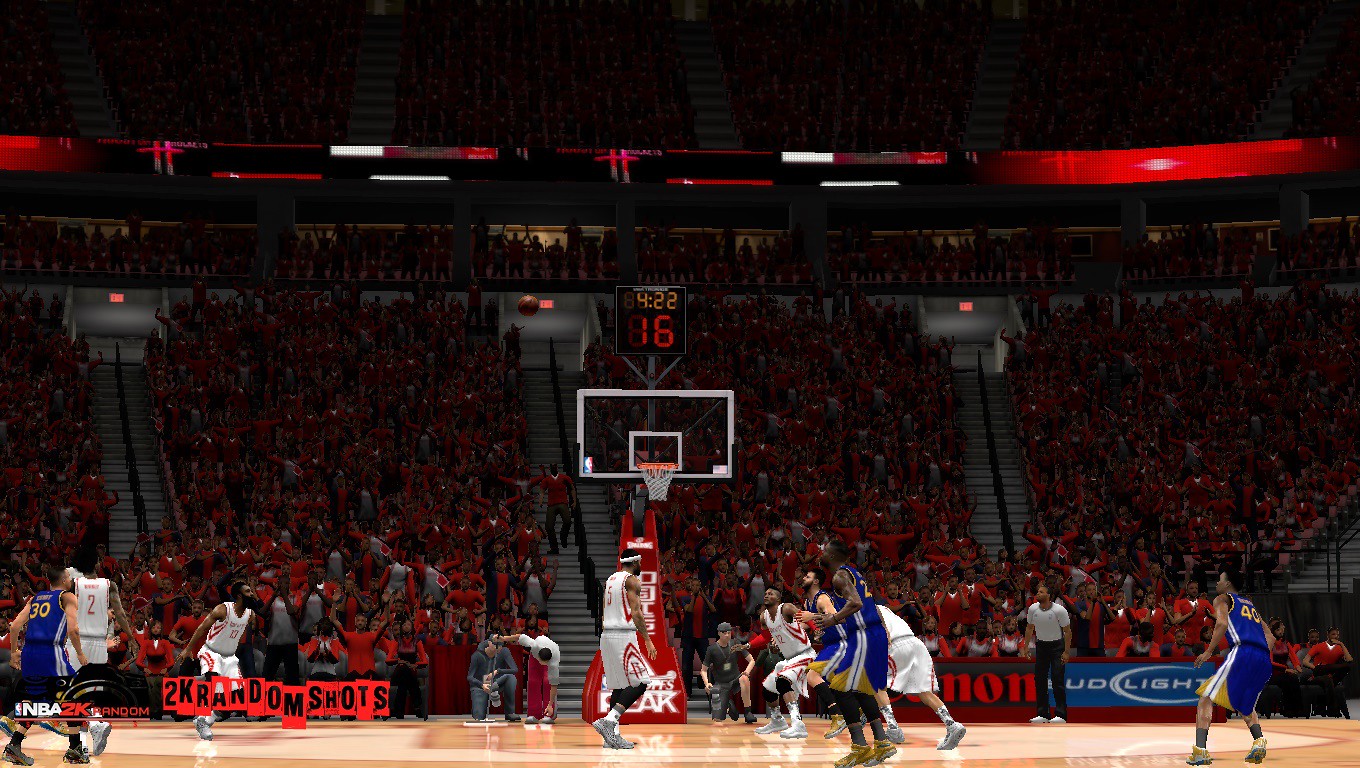In this image, an NBA 2K basketball game is in progress, indicated by the game interface visible in the bottom left-hand corner. The two opposing teams are distinguished by their uniforms: one team is dressed in red and white, while the other dons blue and gold. The game clock at the top of the screen shows 4 minutes and 22 seconds remaining. Additionally, a secondary clock displays 16 seconds, possibly indicating the shot clock. The stadium appears to be quite full, with a significant number of fans in the crowd wearing red to show their support for the red team. The atmosphere suggests a lively and engaging game, with fans deeply invested in the action on the court.